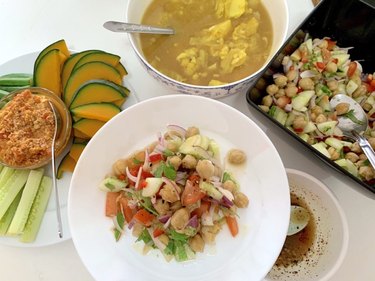The image showcases a richly detailed spread of diverse foods arranged on a table. At its center is a white plate showcasing a colorful chickpea salad, garnished with cucumbers and red onions. Adjacent to this, a circular white plate holds a slice of kombucha squash, contributing to the array of flavors. Prominently featured is a black takeout container also filled with the vibrant chickpea salad. Among the assorted items, multiple white plates and bowls are visible. One white bowl contains a brown, curry-infused soup with a mustard hue, indicative of its flavorful spice content. Scattered across the table are vegetables, including celery, avocados, and leafy greens, along with a clear bowl of salsa dip. Several silver spoons are placed within the bowls, suggesting the meal is ready to be enjoyed. The overall presentation is inviting and visually appealing, highlighting the tasty and varied selection of food.